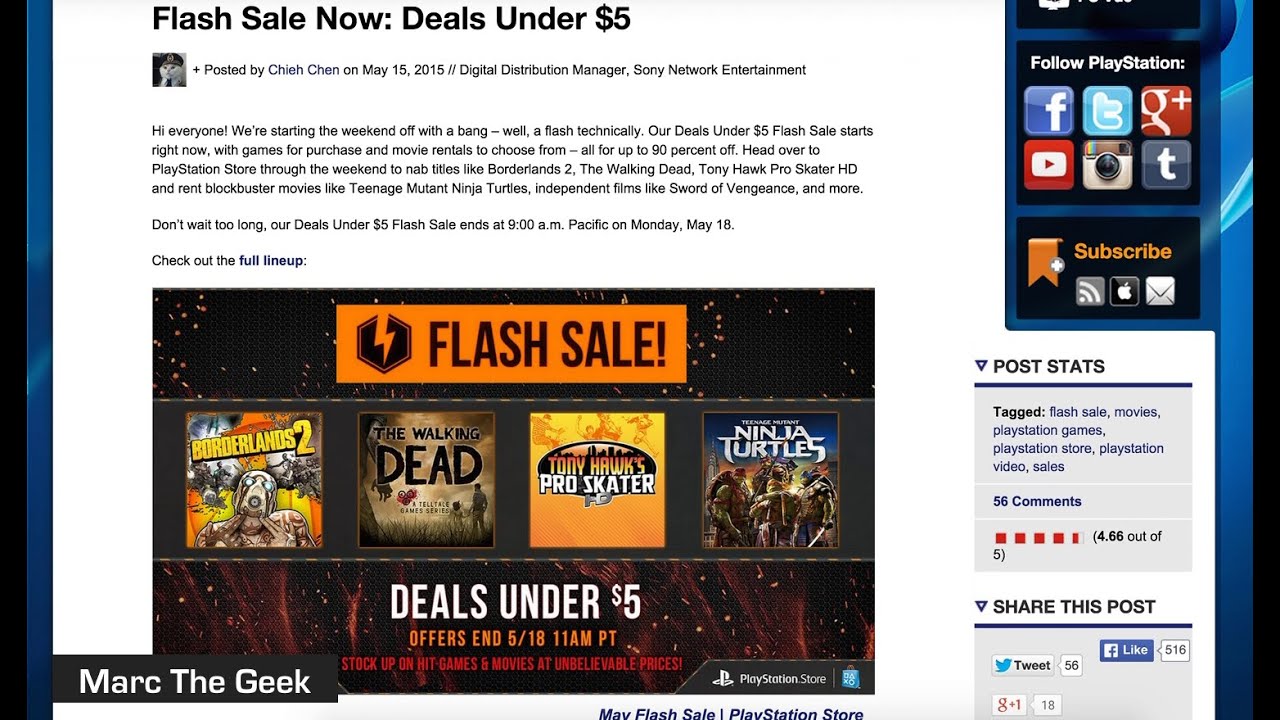This image is a detailed screenshot from a website announcing a "Deals Under $5" flash sale. The announcement, authored by Chish Shen, Digital Distribution Manager at Sari Network Entertainment, was posted on May 15, 2015. The promotion, which kicks off the weekend, offers a variety of highly discounted items available through the PlayStation Store. The text in the screenshot reads:

"Hi everyone, we're starting the weekend off with a bang—well, a flash technically. Our deals under $5 flash sale starts right now, offering up to 90% off on games for purchase and movie rentals. Head over to PlayStation Store through the weekend to nab titles like Borderlands 2, The Walking Dead, Tony Hawk Pro Skater HD, and movies like Teenage Mutant Ninja Turtles, as well as independent films like Sword of Vengeance, and more. Don’t wait too long; our deals under $5 flash sale ends at 9 a.m. Pacific on Monday, May 18. Check out the full lineup."

The phrase "flash sale" is prominently featured in a bold orange box with black letters, and a selection of the discounted deals is visible below.